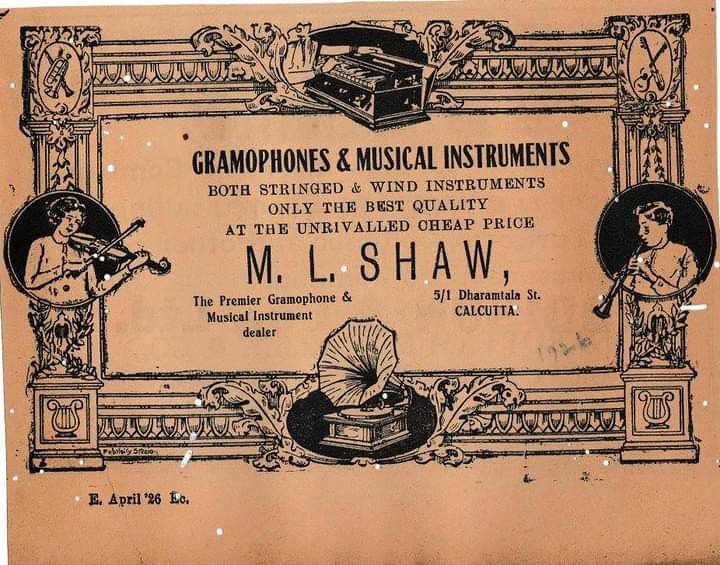This vintage advertisement, dated April 26, 1926, from the company M. L. Shaw, features a beautifully detailed and regal frame around the text and illustrations, reminiscent of a museum exhibit. The aged paper has a brown, peachy hue, suggesting its considerable age. Within the ornate borders, two musicians are depicted in circular portraits—a woman playing a violin on the left and a young boy playing a clarinet or an oboe at the bottom. A grand piano is prominently positioned at the top center, while an old-fashioned gramophone with a large horn speaker occupies the bottom of the image. The advertisement is textually rich, written in black ink, clearly stating: "Gramophones and musical instruments, both stringed and wind instruments, only the best quality at the unrivaled cheap price. M. L. Shaw, the premier gramophone and musical instrument dealer, 5-1, Darmesha Street, Calcutta."